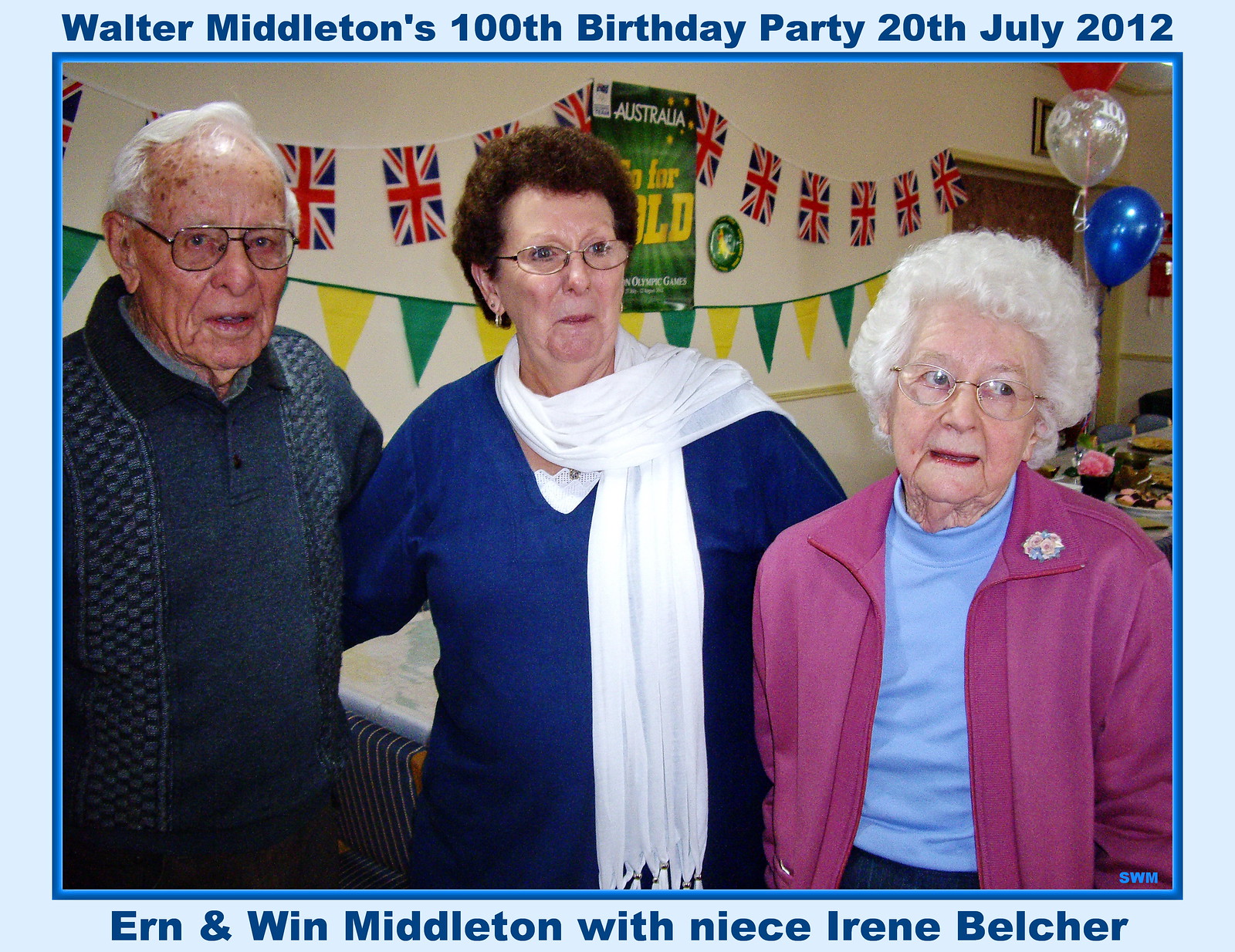This photo captures a festive scene at Walter Middleton's 100th birthday party on July 20, 2012, framed with a blue border. The top of the image is labeled "Walter Middleton's 100th Birthday Party 20th July 2012," while the bottom reads, "Earn and Wynn Middleton with niece Irene Belcher."

From left to right, the first person is an elderly gentleman with white hair, glasses, and a blue sweater. In the center stands Irene Belcher, who appears younger than the other two. She has dyed brown hair, wears glasses, a blue shirt, and a white scarf draped over her shoulder. On the right is Wynn Middleton, an older woman with white hair, a pink coat, and a blue shirt.

The trio stands in front of a wall adorned with festive UK flags and banners alternating between yellow and green. The background also features balloons and what looks to be food laid out on a table, adding to the celebratory atmosphere. Their varied facial expressions add a touch of personality to the joyous moment captured in the photograph.